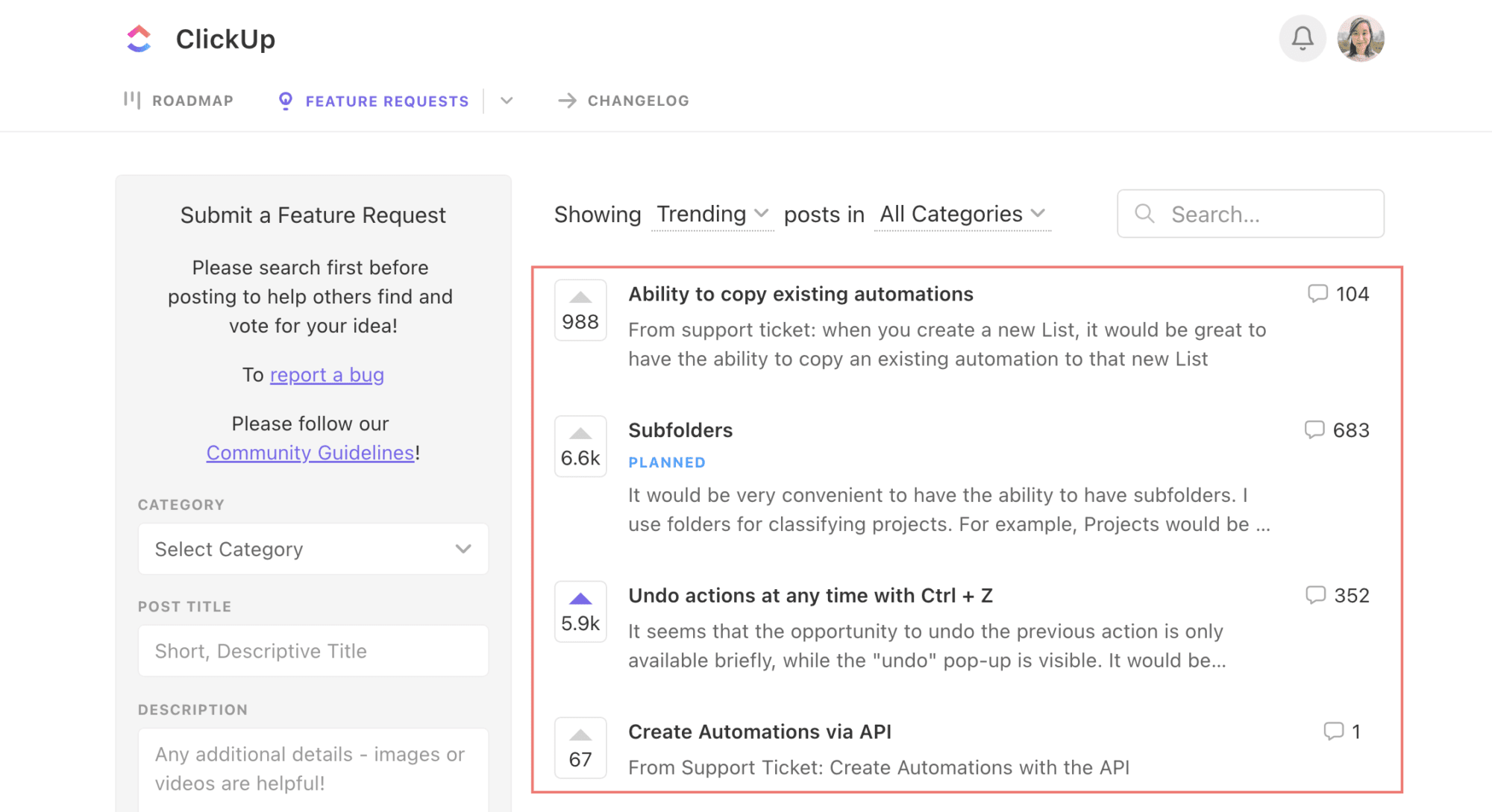### Detailed Caption for the ClickUp Web Page:

#### Top Navigation Bar:
- **Logo Area:**
  - The ClickUp logo is positioned at the top left corner.
  - The logo features "ClickUp" in black lettering with a capital 'C'.
  - To the left of the text is an icon consisting of a red upward triangle and a blue horizontal curve beneath it.

#### Right Corner:
- **Notifications and User Image:**
  - A gray circle housing a black or gray bell icon.
  - Next to the bell icon is a circular user image of a girl with a fair complexion and long blonde hair.

#### Primary Navigation Tabs:
- **ROADMAP:** 
  - Displayed in all caps using gray lettering.
  - Accompanied by three lines of varying lengths (medium, small, large) to its left.
- **FEATURE REQUEST:**
  - Written in all caps with blue lettering.
  - To the right of this tab is a vertical gray line and a small downward gray arrow.
- **CHANGE LOG:**
  - In all caps, gray lettering.
  - A gray arrow pointing to the right is positioned to the right of this label.

#### Main Content Sections:
- **Submit a Feature Request Section:**
  - A gray rectangular area is labeled "SUBMIT A FEATURE REQUEST" with 'S', 'F', and 'R' capitalized.
  - Below, instructions read: "PLEASE SEARCH FIRST BEFORE POSTING TO HELP OTHERS FIND AND VOTE FOR YOUR IDEA," with 'PLEASE' and 'TO' being capitalized.
  - Underlined text in gray, "REPORT A BUG," appears in a purple font.
  - Further below, it instructs: "PLEASE FOLLOW," with 'PLEASE' capitalized.
  - Next, "COMMUNITY GUIDELINES!" is noted, where 'C' and 'G' are capitalized, and underlined in purple.

- **Category Selection Area:**
  - The label "CATEGORY" appears in all caps, gray lettering.
  - A white rectangular box with a drop-down button on the left offers the option to "SELECT CATEGORY," in black, capitalized letters.
  - "POST TITLE" is displayed in all caps, with a white rectangular box below it labeled "SHORT DESCRIPTIVE TITLE," also all in caps.
  - Following this, "DESCRIPTION" in all caps leads into a white rectangular box inviting additional details, starting with "A" capitalized, detailing that images or videos are helpful.

#### Right-Hand Sidebar:
- **Trending Posts Display:**
  - A section beginning with "SHOWING TRENDING" in black lettering and a downward arrow.
  - Followed by "POSTS IN" and a drop-down for "ALL CATEGORIES," each capitalized.
  - This section has light gray lines underneath it with a SEARCH BAR captioned "SEARCH…" with a magnifying glass icon to the left within a gray border box.

#### Feature Requests Listings:
- **First Entry (988 votes):**
  - In a red rectangular box with "988" in black inside a gray border box with up/down arrows.
  - The title reads "ABILITY TO COPY EXISTING AUTOMATIONS," in capital letters, and below, in gray: "FROM SUPPORT TICKET; when you create a new list, it would be great to have the ability to copy an existing automation to that list."
  
- **Second Entry (6.6K votes):**
  - The title "SUBFOLDERS" in blue lettering, "PLANNED" status, and details below in gray: "It would be very convenient to have the ability to have subfolders. I use folders for classifying projects, for example, projects…"
  
- **Third Entry (5.9K votes):**
  - "UNDO ACTIONS AT ANY TIME WITH CONTROL + Z" with 'UNDO,' 'CONTROL,' and 'Z' capitalized.
  
- **Fourth Entry (6.7 votes):**
  - "CREATE AUTOMATIONS VIA API FROM SUPPORT TICKET" in black capitalized letters.

Each post has a gray border box on the right corner with a number inside, representing comment counts.